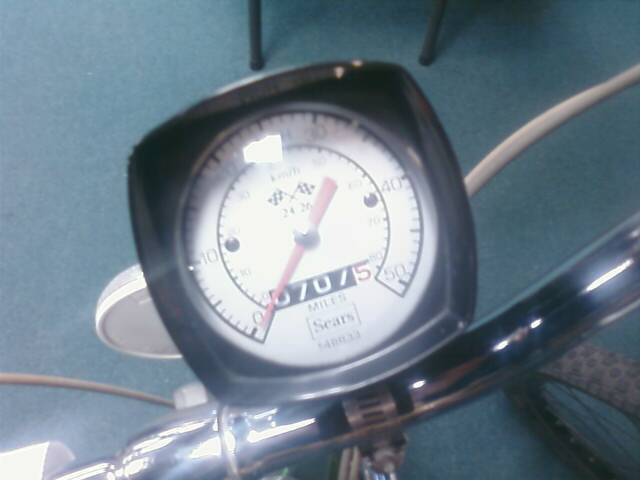The image depicts a vintage odometer on what appears to be a dirt bike or motorbike, set against a slightly blurry and old-fashioned backdrop. At the center is a large, square, black panel that houses the odometer. The odometer itself is circular, with a white face adorned with black numbers and lines, and a red needle pointing out the readout. The scale ranges from 0, with discernible increments including 10, possibly 30, 40, and 50, though some numbers are obscured by glare. Positioned above the needle are two crossed checkerboard flags, symbolizing racing or completion. Below this emblem, the odometer reading displays '07075' miles. The brand 'SEARS' is inscribed beneath it. Surrounding the odometer, parts of the bike, such as silver handlebars and a portion of a black tire in the lower right corner, are visible. Additionally, a white light can be seen behind the odometer. The floor beneath the bike is a peculiar greenish-teal hue, the exact material unknown, adding to the image's vintage aesthetic.